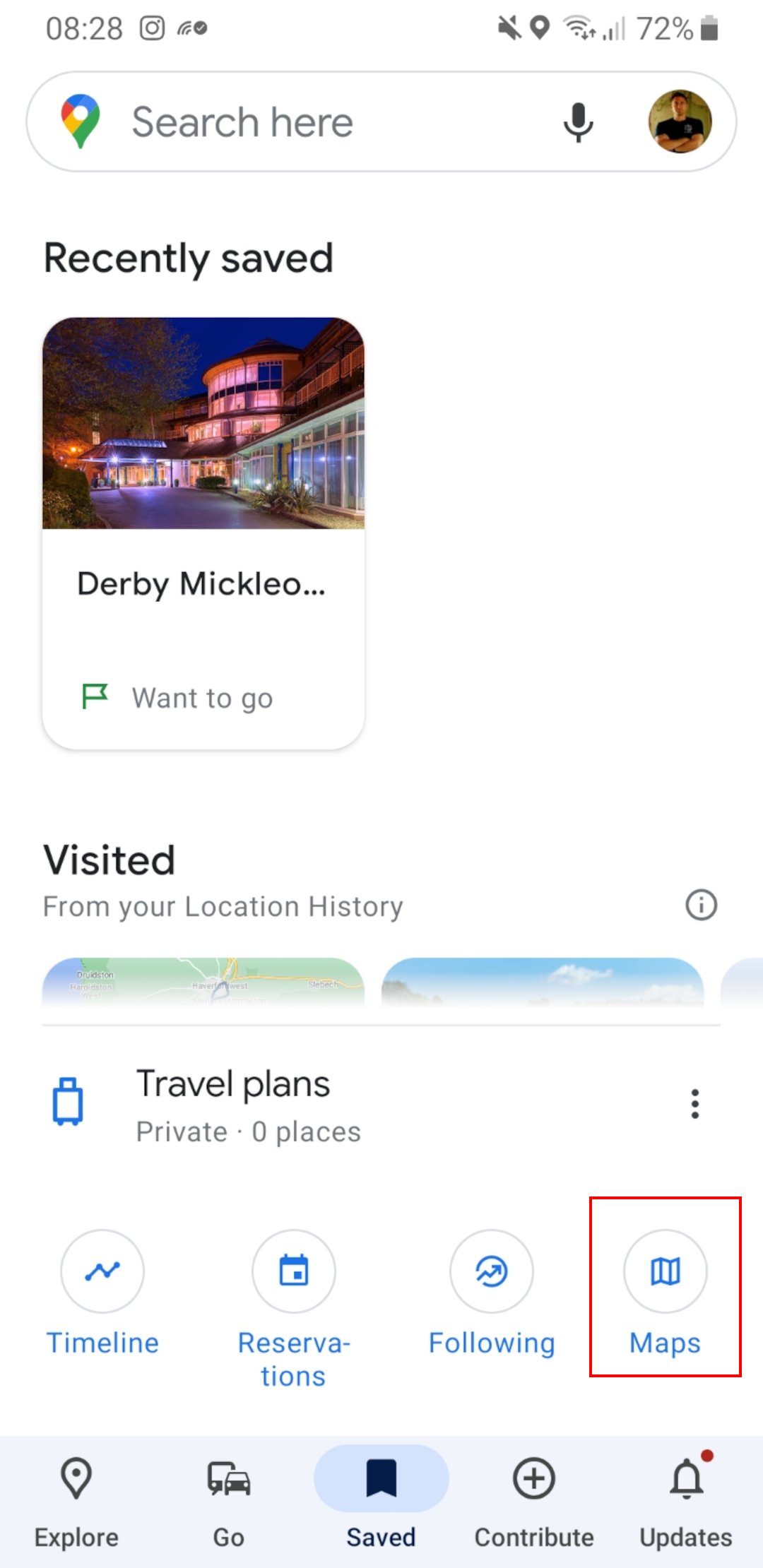This image is a screenshot of the Google Travel section on a cell phone, set against a white background. At the top, there is a prominent search bar featuring a pin drop icon in Google colors to the left, accompanied by gray text that says “Search here.” To the right of this text, a microphone icon is present, and the user's profile picture is positioned at the far right edge of the search box.

Beneath the search bar, on the left side, bold black text states “Recently saved.” Below this, a thumbnail image appears with a relevant photo at the top. Underneath the photo, black text partially reads "Derby McLeo," followed by an ellipsis indicating the rest of the word is truncated. Adjacent to this is a small flag icon to the left, and the phrase "Want to go" in small gray letters to the right.

Further down, the category "Visited" is presented in large black letters. Below this category, small gray text reads "From your location history." Visible are the top edges of additional thumbnails, suggesting that more content would be revealed upon scrolling.

At the bottom left, there is a blue suitcase icon followed by the text "Travel plans" in black. Similarly, “Private” and “Zero places” are displayed in small gray letters beneath it. The very bottom of the search interface contains four boxed options labeled "Timeline," "Reservations," "Following," and "Maps." Notably, the "Maps" option is highlighted with a red box, which appears to be a later edit made to the photo.